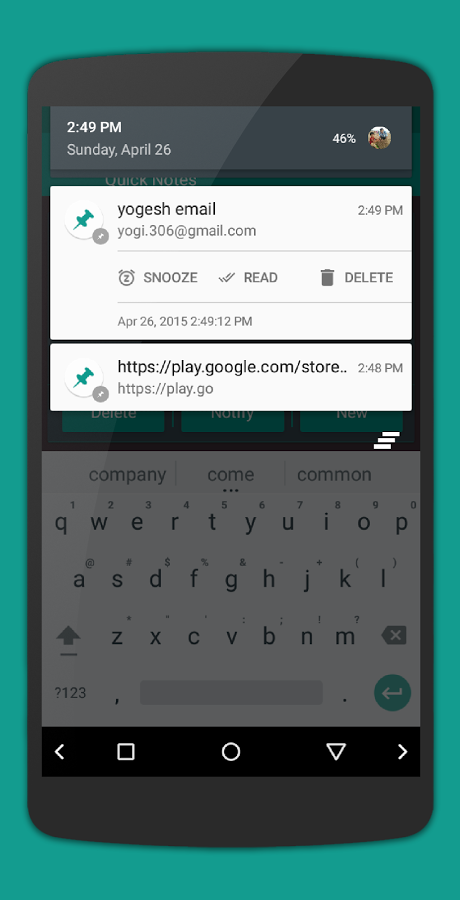The image, captured in portrait mode, showcases a digital device set against a teal, greenish-teal background which frames the device prominently. The device appears to be a tablet or a vertically compressed smartphone. At the top of the screen, the device display reads "2:49 PM, Sunday, April 26th." To the top right is the battery icon showing a 46% charge. Next to it, there is a small, round user profile photo.

A white text box dominates the upper segment of the screen, which contains the text:

"Yogesh Email,
2:49 PM,
yogl.306@gmail.com"

Adjacent to this text is a blue pushpin icon. Below this section, there is a horizontal line followed by a row of three clickable icons labeled "Snooze," "Read," and "Delete." The "Snooze" option features an alarm clock icon with a 'Z,' the "Read" option has double check marks, and the "Delete" option displays a trash can icon. Beneath this row, another thin line appears.

Further down, the screen displays the following timestamp: 

"April 26th, 2015, 2:49 and 12 seconds PM."

This is followed by a thick gray divider line. Below it, the text "HTTPS" (indicating a secure URL), along with "secureplay.google.com" (a Google Play Store address), is displayed next to another blue pushpin icon and a timestamp reading "2:48 PM."

The bottom half of the screen contains a full QWERTY keyboard layout. Above the keyboard, autofill suggestions are shown, displaying the words "Company," "Come," and "Common," indicating the user was likely in the process of typing.